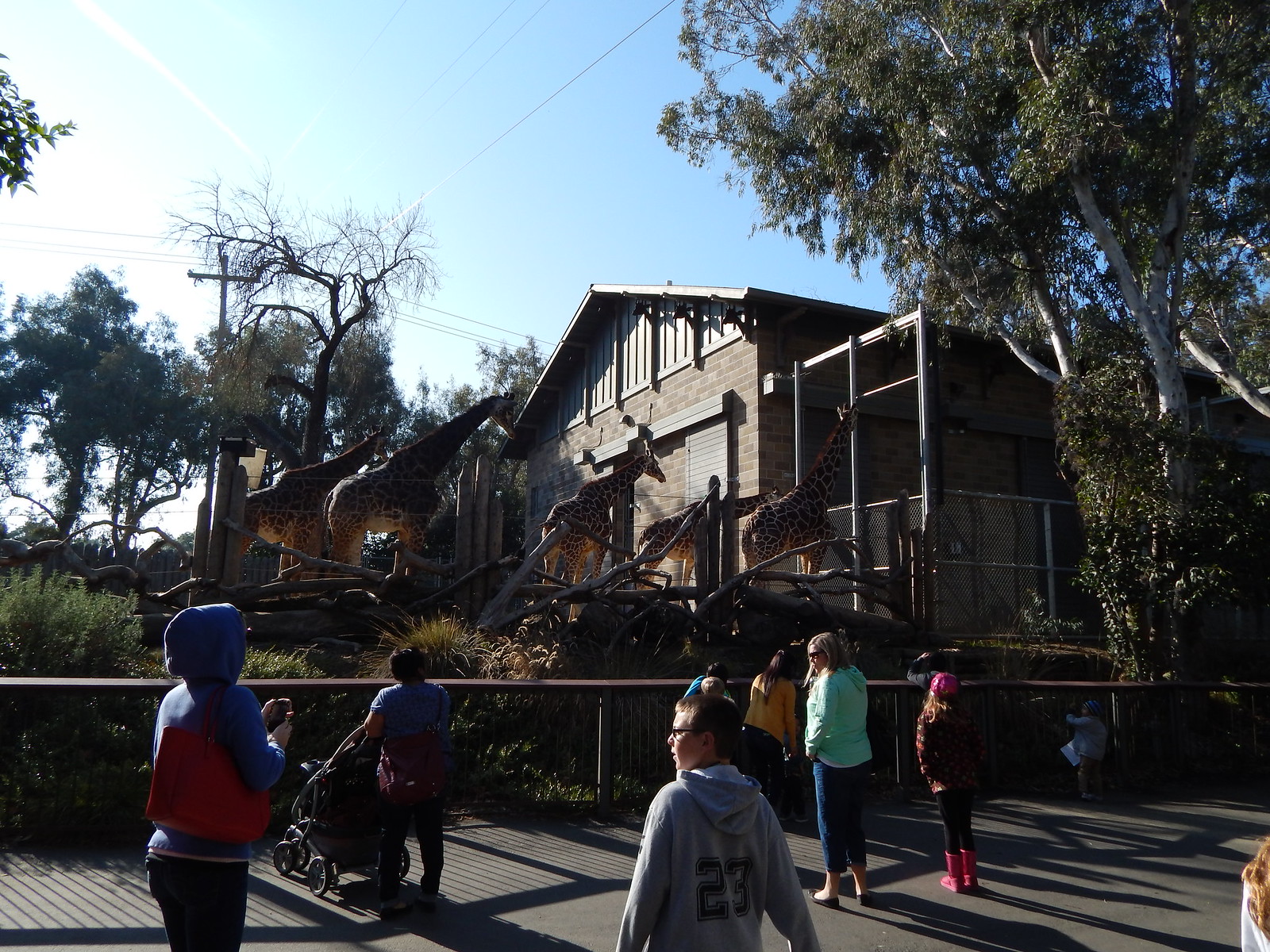The image captures a cold day at a zoo, with five giraffes near a large brick building, possibly a shed for their enclosure. The giraffes, towering and stately, are all moving in the same direction with their heads turned away from the camera. The scene is framed with numerous trees: a tree on the right, one directly behind the giraffes, and another on the top left indicated by visible leaves. A substantial wire fence surrounds the giraffe enclosure, while a secondary wooden fence directs the visitors, keeping them a safe distance away. Approximately eight people are visible, some in coats, suggesting chilly weather. Among the visitors is a lady with a stroller, all standing on a wide concrete pathway. Power lines and a pole are also visible, adding an urban element to the otherwise natural setting. The entire scene is orderly and structured, with the fences ensuring clear boundaries between the giraffes and the zoo guests.